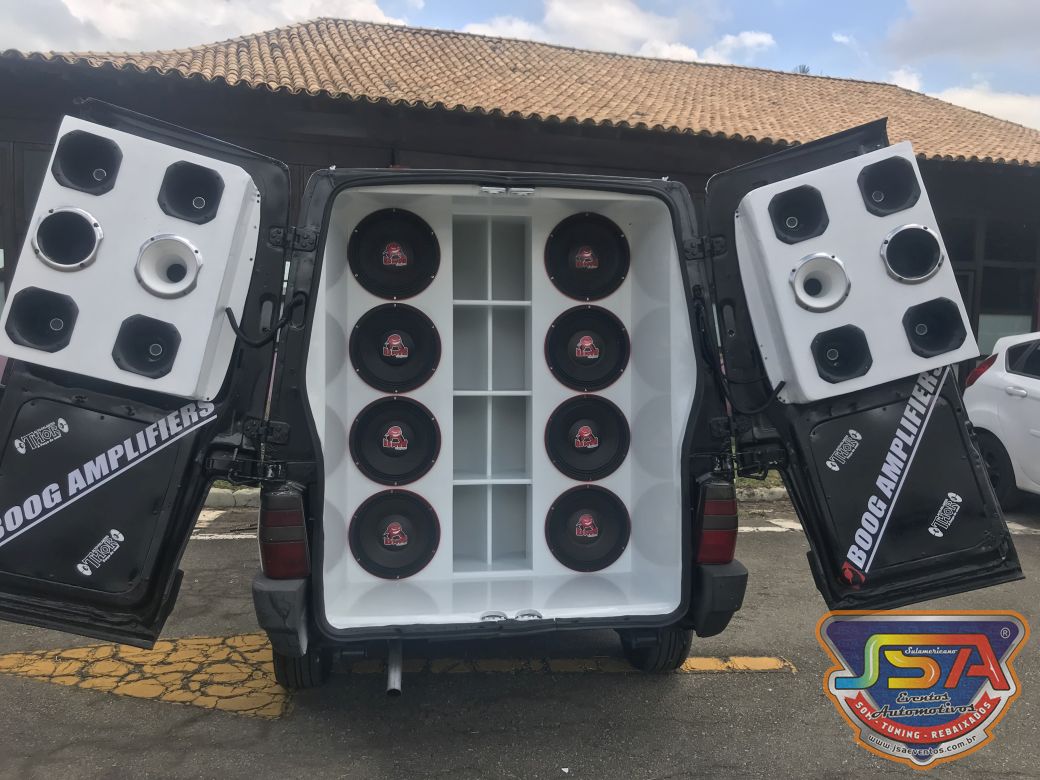In a bustling parking lot with cracked black asphalt and a yellow directional arrow, a black minivan stands out with its back doors wide open, showcasing a powerful sound system. The interior and doors of the minivan are outfitted with an array of speakers. Inside the van, two columns of four round speakers each are neatly installed on a white background. The open doors reveal three rows of two square or round speakers per door, also on a white backdrop with a diagonal white line and the words "Boog Amplifiers" prominently displayed. A colorful logo rendered in shades of red, yellow, green, and blue sits at the lower right corner, though its details are hard to decipher. The scene is complemented by a tiled roof building reminiscent of Spanish colonial architecture in the background and a white SUV parked nearby under a blue sky with a few wispy clouds.